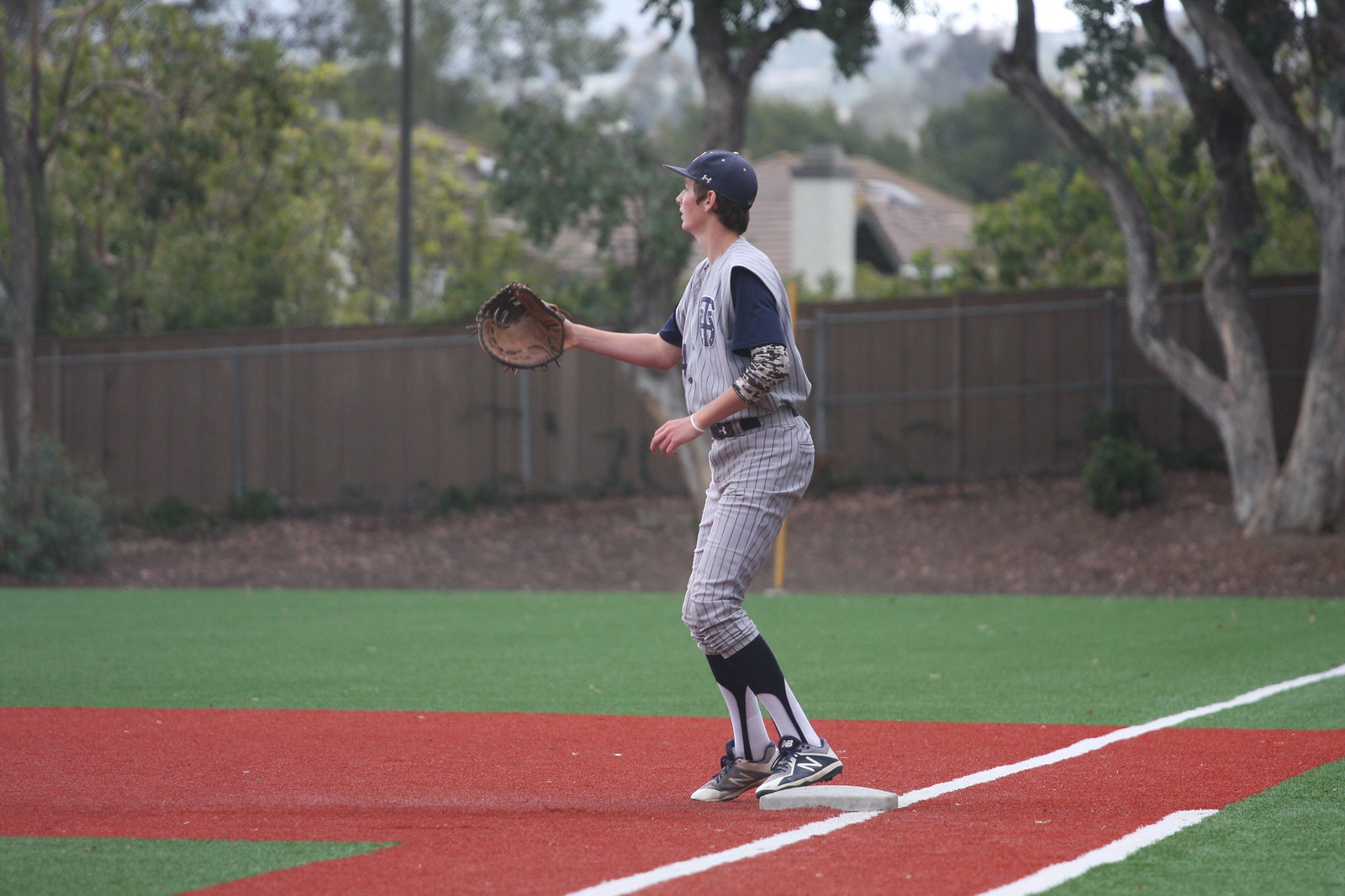The image captures a detailed scene on a residential-style baseball field where a first baseman, clad in a gray uniform with distinctive dark blue pinstripes and blue sleeves, stands. The player is poised, with one foot planted on the first base bag and the other just off it, his left-handed glove outstretched to his right side at chest level, ready to catch an incoming throw. He wears a black or navy cap, black or dark blue stirrups over white socks, and New Balance shoes. Additional attire includes an elbow pad, a white wristband, and a long-sleeve shirt beneath the uniform. The field itself features green AstroTurf grass with red-colored base paths outlined by crisp white stripes. In the background, right field to part of center field is visible, revealing a unique arrangement of trees growing directly in the outfield, with a wooden fence beyond them. This fence appears only partially functional, giving the park a distinct residential feel, further accented by houses and more trees situated behind the fence.